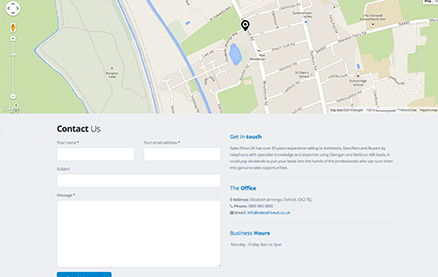The image appears to be a screenshot from a computer interface. The top half of the image features a map with a black pin indicating a location near a small body of water. Due to the low resolution, the street names and finer details on the map are illegible. 

Below the map, the bottom half of the image has a light gray background and contains a "Contact Us" section. This section includes text boxes labeled for the user's name, email address, subject, and message. To the right of these text boxes, the text "Get in Touch" appears in blue, accompanied by a paragraph that is too blurry to decipher.

Following this, there is a segment titled "The Office," which lists an address, phone number, and email address, although the specifics are obscured by the image's blurriness. Additionally, there is a "Business Hours" section indicating operating days from Monday through Friday, but the exact hours cannot be read.

At the bottom of the "Contact Us" section, there is a blue submit button, recognizable by its size and color, despite the absence of any visible text within it. The map itself features zoom in and out functionalities located on the left-hand side.